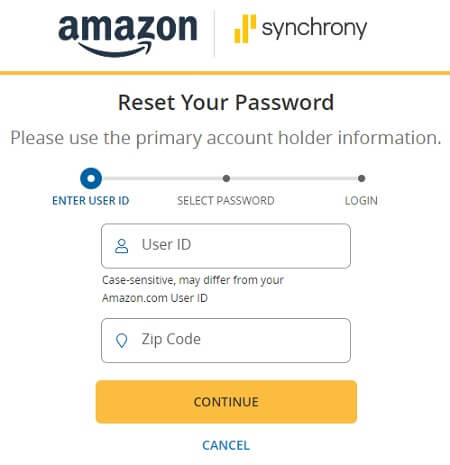The image depicts a login page associated with Amazon or an Amazon affiliate, prominently featuring an Amazon logo on the top left and "Synchrony" to the right of the logo. Below these, centrally positioned, is the heading "Reset Your Password." A directive underneath instructs users to "please use the primary account holder information." 

A vertically-oriented timeline graphic is displayed, illustrating three steps: "Enter User ID," "Select Password," and "Login." The first input field is labeled "User ID," followed by another field labeled "ZIP Code." 

Between the User ID and ZIP Code fields, there is a note in gray text that reads, "Case-sensitive, may differ from your amazon.com User ID."